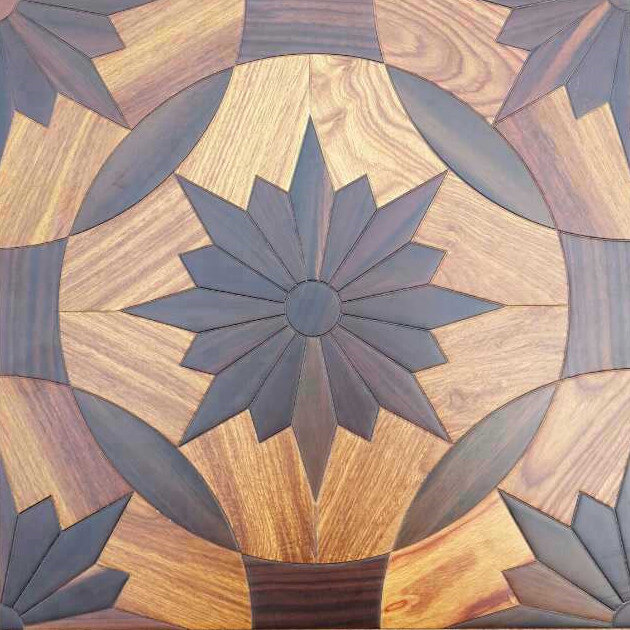The image depicts a detailed wooden engraving with intricate geometric patterns. The entire piece is a complete square, primarily showcasing various shades of brown, from light beige to dark brown, highlighting the natural beauty of the wood. Central to the design is a sunburst or starburst motif, radiating from the middle of the square. Surrounding this central burst is a circle, which seamlessly integrates with the rest of the pattern.

On the bottom corners of the piece, carved elements resembling arrow sprouts or petals are carefully mirrored on both sides, adding to the intricate and symmetrical design. These elements flow into arc shapes that guide the eye back to the central motif. The craftsmanship showcases a Concordant order, with every detail on the left mirrored on the right, resulting in a balanced and harmonious composition.

This woodworking detail, devoid of any textual elements, emphasizes the ornate nature of the woodwork, with the varied shades of brown creating depth and contrast within the design.